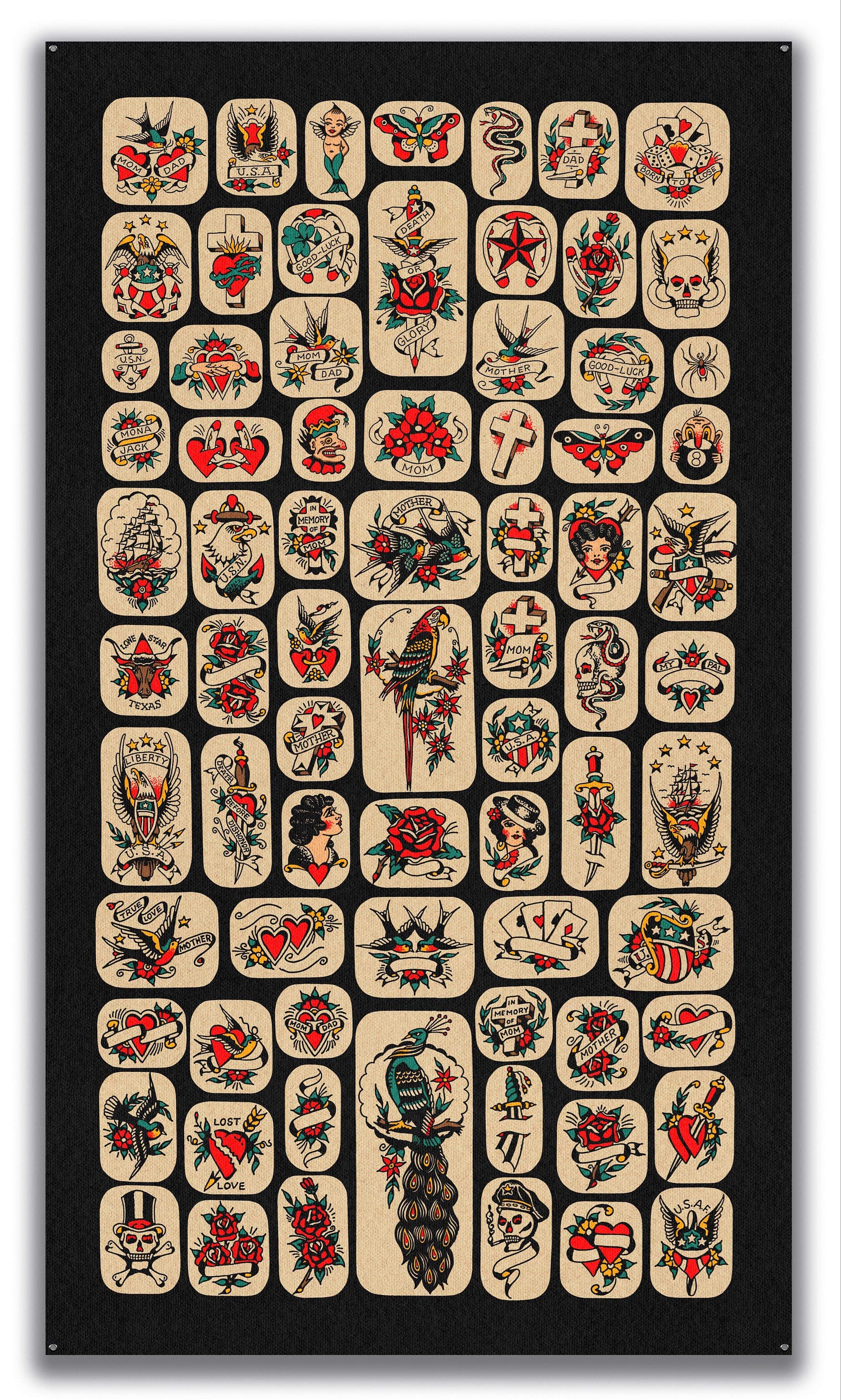The image displays a large, vertically oriented sheet showcasing a rich collection of traditional tattoo flash designs against a cream-colored background. Each individual tattoo design is meticulously cut out and affixed to a black surface using thumbtacks at all four corners, highlighting the intricate details and vibrant colors of the artwork. The designs are mostly small squares and rectangles with some larger ones positioned centrally. Dominant colors include candy apple reds, greens, blacks, grays, and yellows, typical of Sailor Jerry-style tattoos. The collection features a variety of iconic motifs such as hearts, some labeled “Mom” and “Dad”, snakes, crosses, and eagles. Additional elements include ribboned banners, playing cards, skulls, women's faces, and flowers. Noteworthy designs among the collection are a bald eagle with stars, a skull with wings, a butterfly, a bull with “Lone Star, Texas”, a sword with a rose, a peacock, a horseshoe with a flower, a spider, and a Liberty, USA shield. The image is well-lit, ensuring every design is prominently visible, showcasing the traditional tattoo artistry in vivid detail.